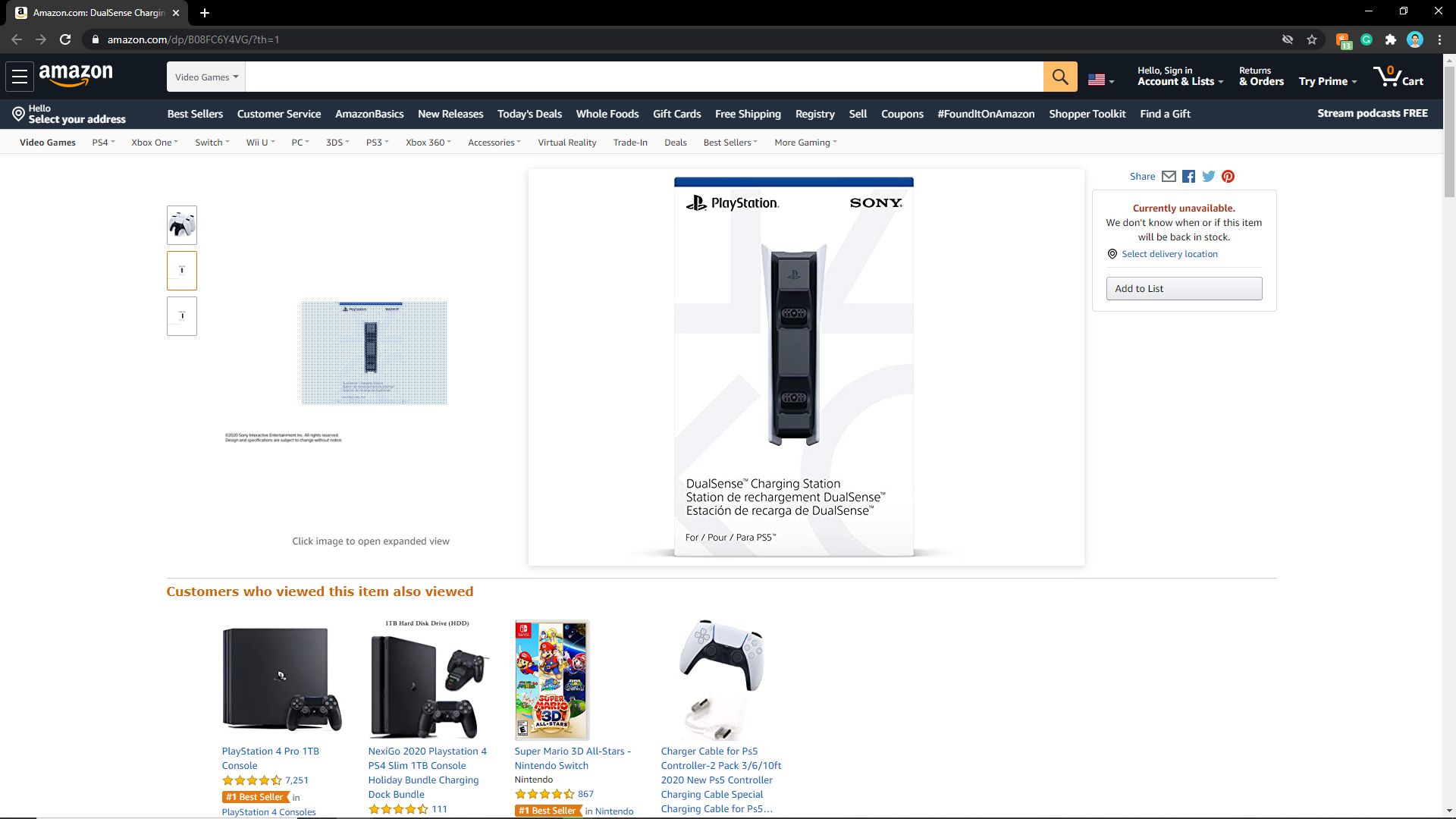The screenshot captures an Amazon.com webpage, open in a web browser as evidenced by the single tab on the top left labeled "amazon.com." The browser's address bar shows the URL beginning with "amazon.com," followed by additional code. In the upper right corner of the browser window, there's a small profile picture that is too indistinct to identify, along with some adjacent icons.

Centered prominently at the top of the Amazon page is the iconic Amazon logo, featuring the word "Amazon" in white, underlined by a yellow arrow curving from the letter "A" to the "Z." Just below the logo is a search field accompanied by a drop-down menu on its left. The gray drop-down menu displays "Video Games" in black text. The search field itself is blank and white, with a golden square containing a black magnifying glass icon on its right end for initiating searches.

Immediately to the search field's right is an American flag icon, coupled with a drop-down menu arrow beside it. To the right of this flag, text reads, "Hello, Sign in Account & Lists Returns & Orders Try Prime," indicating links for signing in, accessing account details, and navigating various service categories. Finally, on the far right, there is a cart icon displaying the number zero, indicating an empty cart.